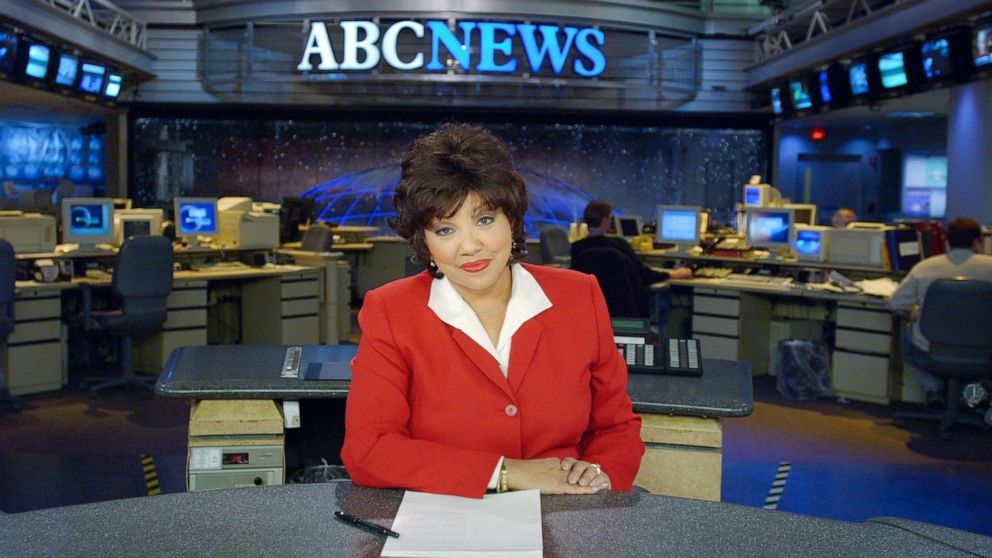In the image, a newscaster with voluminous, slightly curly brunette hair styled into a bun, and bangs kept neatly out of her eyes, sits at the foreground. She has tan skin and is wearing red lipstick. Her outfit consists of a red suit jacket buttoned up and a white collared shirt underneath. She rests her left hand over her right on an oval, gray stone-like desk, where a white piece of paper and a black pen are placed.

Above her, the network logo "ABC News" is prominently displayed, with "ABC" in illuminated white and "News" in lit-up blue. The backdrop features a bustling newsroom with numerous older, thick-screened computer monitors arranged on white desks, accompanied by blue office chairs. A couple of individuals, wearing black or white shirts paired with blue pants, work diligently at their stations, their backs turned to the camera. 

The walls are painted in shades of blue and silver, and several black square TVs are mounted high up, showing various blue, white, and black visuals. There are black garbage cans with clear liners scattered around, and the desks have black strips on the drawers. Behind the newscaster, another gray desk can be seen, framed by the general busy ambiance of the newsroom.